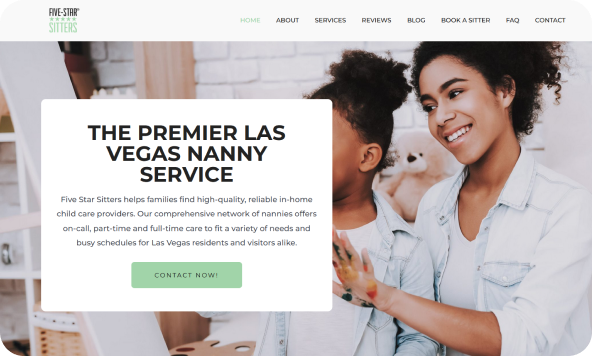In the image, two individuals are featured: an adult woman and a young girl, both dressed in coordinated outfits of denim shirts and white t-shirts. They appear to be in a bright, predominantly white room with white brick walls, accentuated by Langenberger baskets which add a rustic touch to the decor. The environment suggests a comfortable, homey setting. The adult woman's hands are covered in paint, indicating that she has been finger painting with the child, who is presumably under her care. An easel with painting supplies in the background reinforces this activity. The image serves as an advertisement for a premier Las Vegas nanny service, promoting "Five-Star Sitters," a service dedicated to helping families find high-quality, reliable, in-home childcare providers. The service offers a comprehensive network of nannies available for on-call, part-time, and full-time care to accommodate the diverse needs and schedules of both Las Vegas residents and visitors. A green box in the advertisement emphasizes a call to action, urging viewers to "Contact Now."